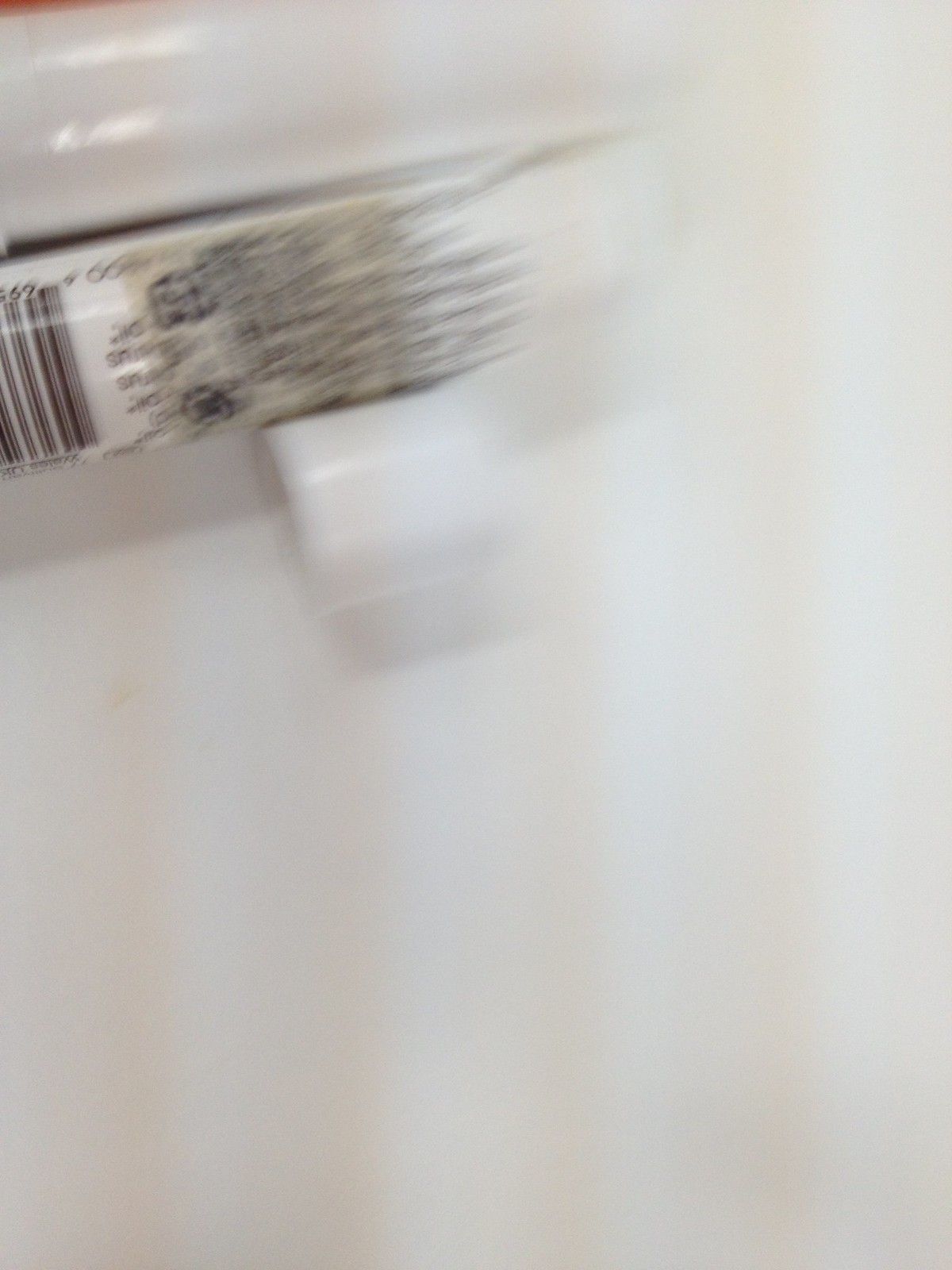This image depicts a very blurry view of what seems to be a label on the side of a white container. The surface of the container is solid white with a pattern of vertical orange stripes, though it is uncertain whether these stripes are a feature of the container or artifacts from the camera itself. In the top left corner of the image, there is a shiny, white item whose details are not clearly discernible. Toward the bottom left of the container, there is a barcode, accompanied by other black text that is too blurred to be read accurately. The overall blurriness of the image makes precise identification challenging.